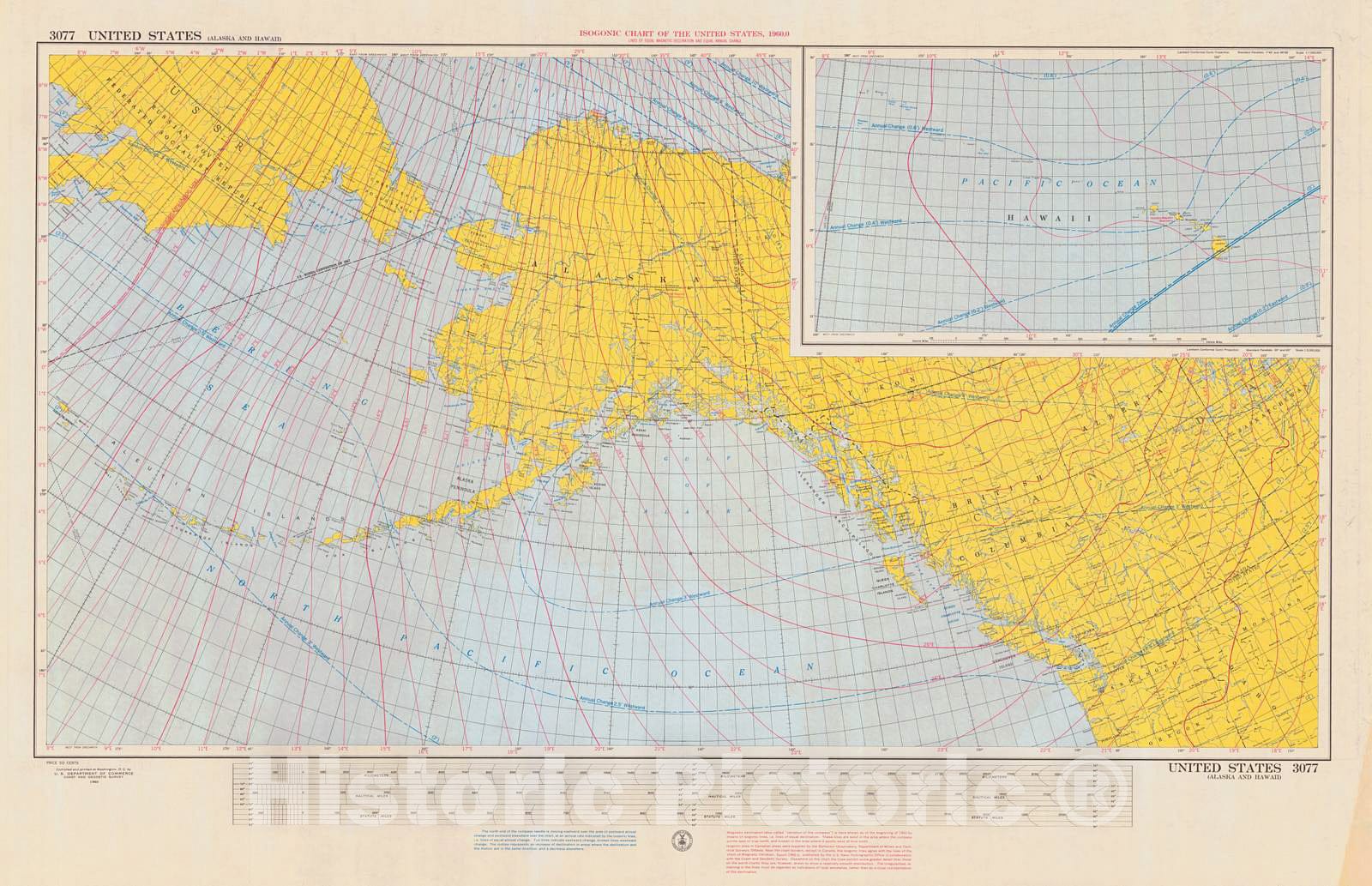The image depicts a detailed, colored map predominantly highlighting Alaska and the northwestern portion of the United States. It features clear demarcations of national borders, major cities, capitals, rivers, lakes, and mountain ranges, each distinguished by various colors. Notably, the map includes compass directions, as well as longitudinal and latitudinal lines, providing geographical context. The background of the map is light blue for oceans and light beige for certain countries, with Alaska prominently labeled next to the USSR on the top left corner of the map. There is a legend at the bottom of the page, although it is small and difficult to read. Additionally, the bottom center of the image bears a watermark that reads "Historic Pictoric." The map is bordered by a very light pinkish-tan frame, and an inset image in the upper right corner offers a zoomed-out view, enhancing the overall detail and context of the showcased geographical region.